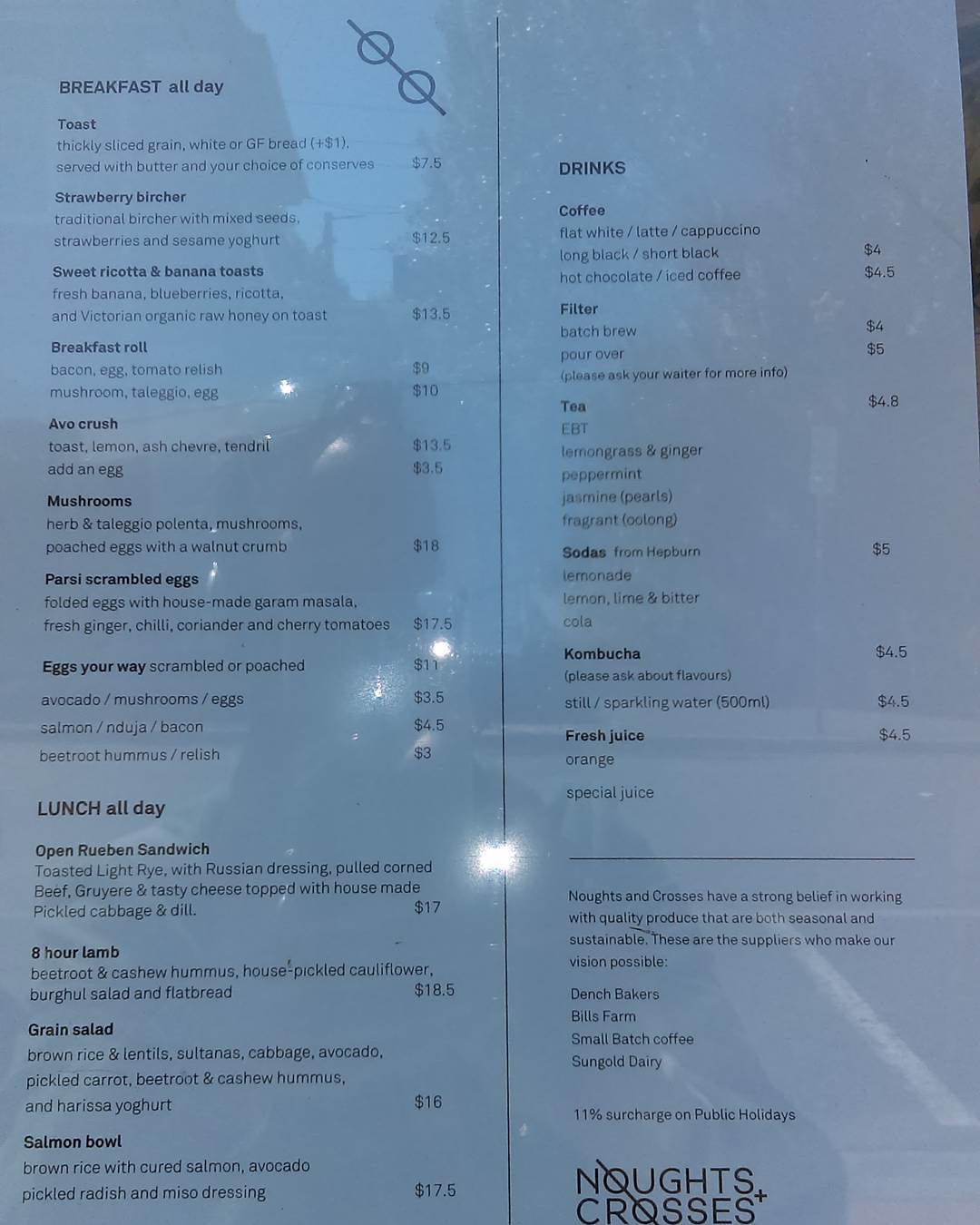This photograph captures a shiny, laminated menu from a local eatery, protected to allow for easy cleaning. The menu is categorized into sections with "Breakfast All Day" at the top, "Lunch All Day" at the bottom left, "Drinks" at the upper right, and "Noughts & Crosses" in a stylized format along with a plus sign towards the bottom right. Additionally, there's an 11% surcharge on public holidays mentioned at the bottom right corner. 

The upper left corner of the menu features breakfast options such as toast, strawberry bircher, sweet ricotta and banana toast, breakfast roll, avocado crush, mushrooms, Persian scrambled eggs, and eggs cooked to order. Lunch offerings displayed include an open Reuben sandwich, eight-hour lamb, grain salad, and a salmon bowl. The drinks section lists coffee, filter tea, sodas, kombucha, and fresh juice.

The photograph also highlights the establishment's dedication to quality and sustainability by showcasing their trusted suppliers: Dench Bakers, Bill's Farm, Small Batch Coffee, and Sungold Dairy. This emphasizes their commitment to using seasonal and sustainable products through partnerships with local businesses.